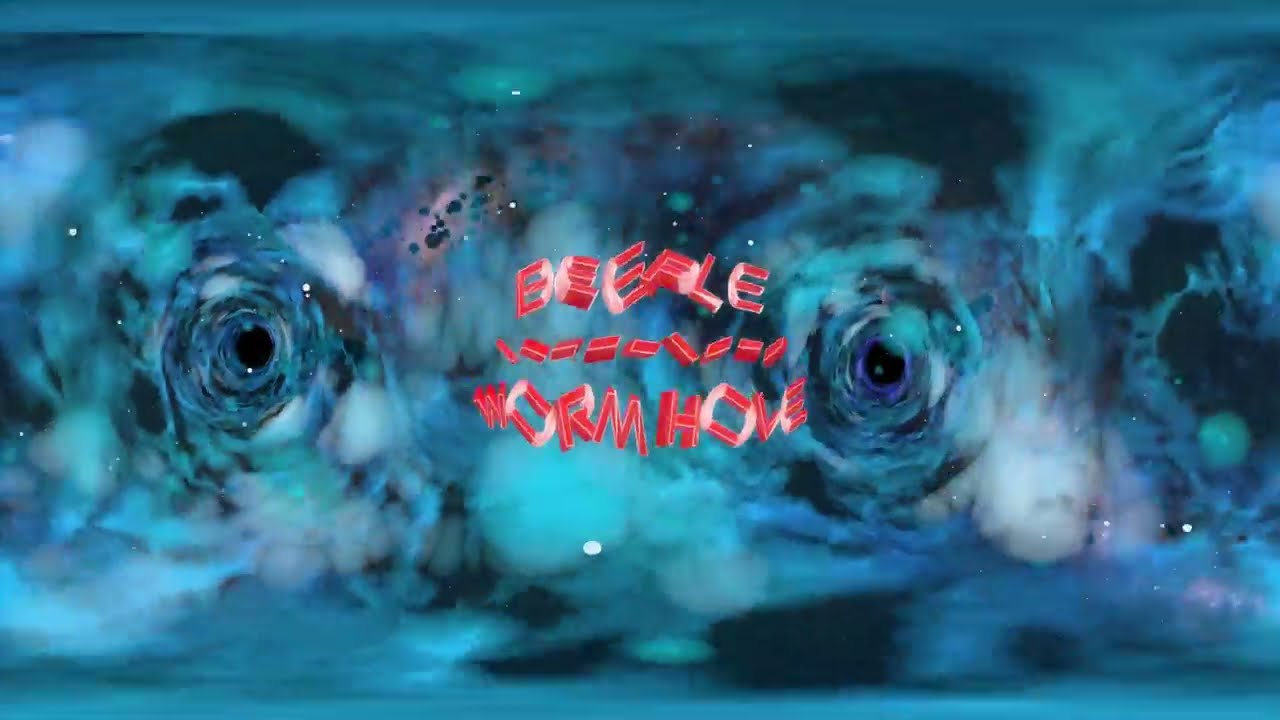The image presents a surrealistic and abstract scene featuring two prominent swirly vortex tunnels on either side, each resembling a black hole or wormhole. The vortices are composed of deep blues, light aquas, teals, and some extremely dark blues that almost appear black, all swirling into dark centers. These tunnels lead into an enigmatic darkness from opposing angles. In the middle of the image, there is an array of broken-up, three-dimensional text in shades of wet red and pink, scattered across three rows. Some of the discernible letters include E, H, W, O, and R, potentially forming fragmented words like "wormhole." The text is twisted and tilted in various directions, making it difficult to read comprehensively. The whole image radiates a cosmic, nebulous aesthetic with abstract lines and shapes that combine to form a complex, dreamlike visual.